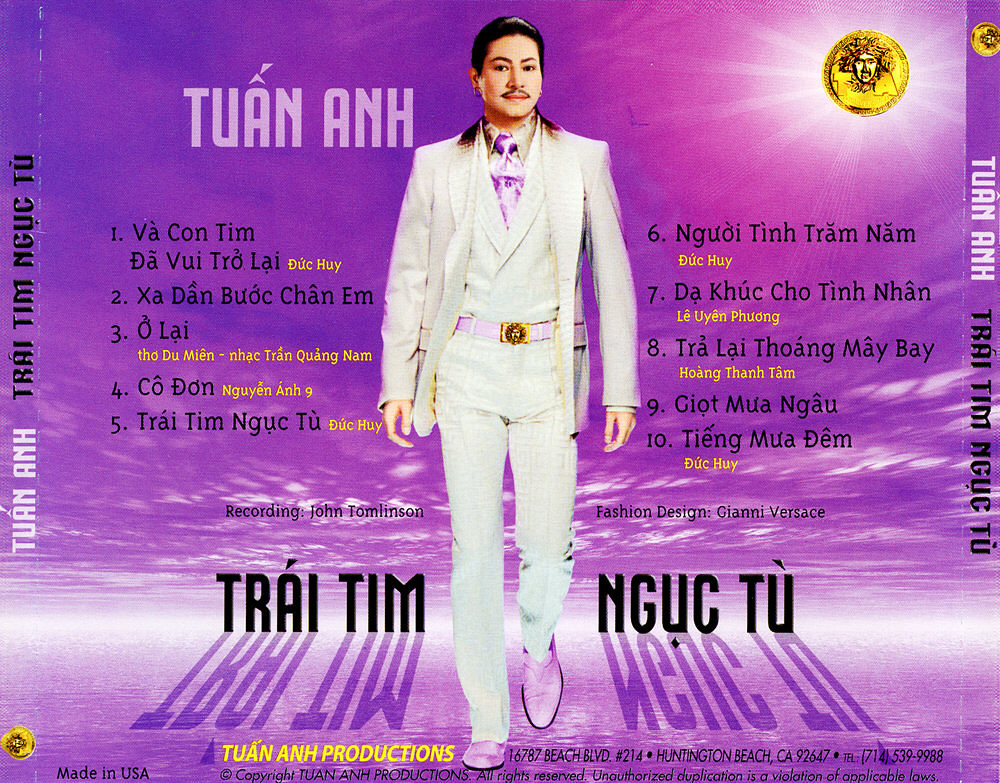This CD cover for the Vietnamese singer Tuan Anh features a digitally rendered image of the artist, who is smiling at the camera from the center of the image. He is elegantly dressed in a lavish three-piece white suit accented with a lilac belt and tie, complementing the album's primarily purple hues. The background depicts shades of purple creating a sky-like scene with a white sun in the right corner. The gold label reads "Tuan Anh Productions," which is repeated on the back cover along with the address 1-678-7 Beach Boulevard, 214 Huntington Beach, California 92647, and a contact number, 714-539-9988. The back artwork lists the titles of 10 songs included in the album, and notes contributions such as fashion design by Gianni Versace and reporting by John Tomlinson. Another label on the spine shows "Tuan A.N.H. Tri-Tim Productions" in white text against a black background.